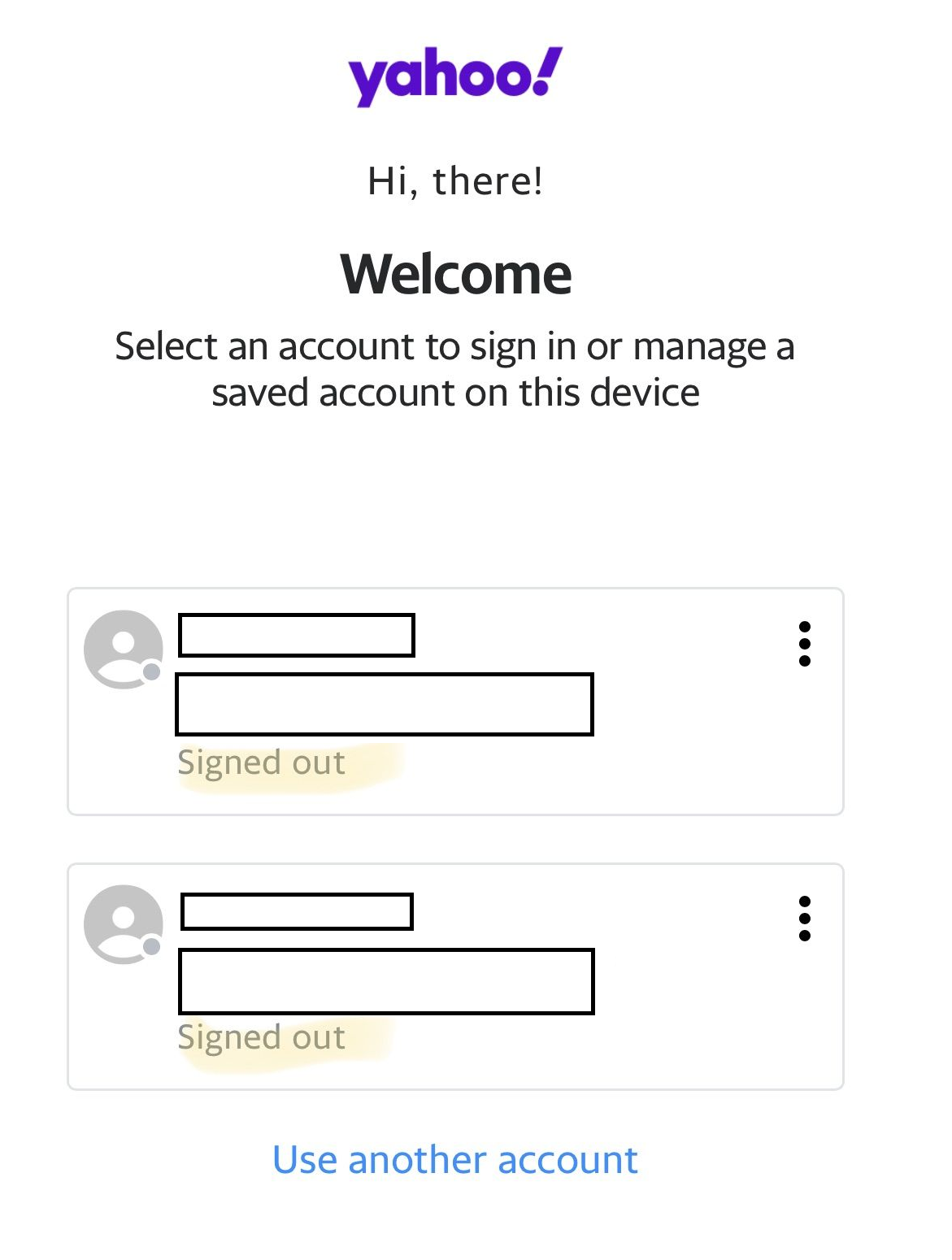The image depicts a Yahoo sign-in screen set against an entirely white background. Centrally positioned at the top, the word "Yahoo" is prominently featured in bold, lowercase, purple letters, with a characteristically tilted exclamation point to the right of the word. Directly beneath this, the text "hi, there!" appears in black type, followed by a larger and bolder "welcome" in black.

Further down, a message in regular black type instructs users to "select an account to sign in or manage a saved account on this device." 

Below the message, there are two distinct sections, each consisting of outlined boxes with light gray borders. In the top left corner of each box, there is a gray circle containing a white person icon. Within each box, there is a small black-outlined rectangular field followed by a larger black-outlined rectangular field. Below this, in gray letters, the term "signed out" is displayed, albeit partially obscured by a yellow smudge. At the top right corner of each gray outline box, three vertical dots are positioned.

Beneath these sections, "use another account" is printed in blue type. The layout indicates that this is a Yahoo sign-in screen, likely showing two previously used accounts that have been signed out, with no specific user identities visible.